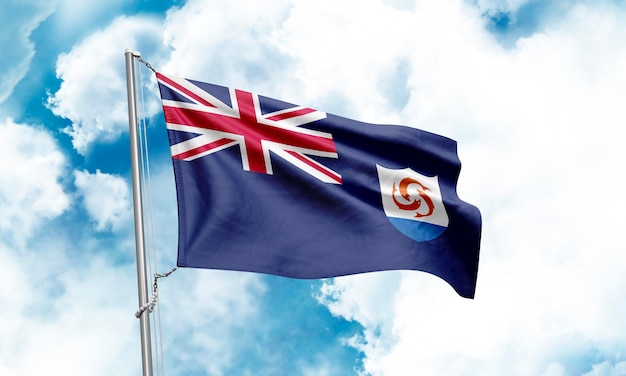The image is a photograph taken outdoors, depicting a flag fluttering heroically on a metallic silver flagpole against a stunning sky backdrop. The flagpole is positioned towards the left side of the horizontally rectangular image, and it's detailed enough to show ropes and attachments. The flag itself is stretched out fully, indicating it's blowing in the wind. It features a dark blue field with the Union Jack occupying the upper left corner. To the right of the Union Jack, there is a shield-shaped emblem that has a white top and a light blue bottom. Inside the shield, three red fish are arranged in a circular or spiral pattern. The background sky is a brilliant blue filled with beautiful, scattered white clouds, illuminated by natural lighting that enhances the overall vibrant and crisp appearance of the scene.